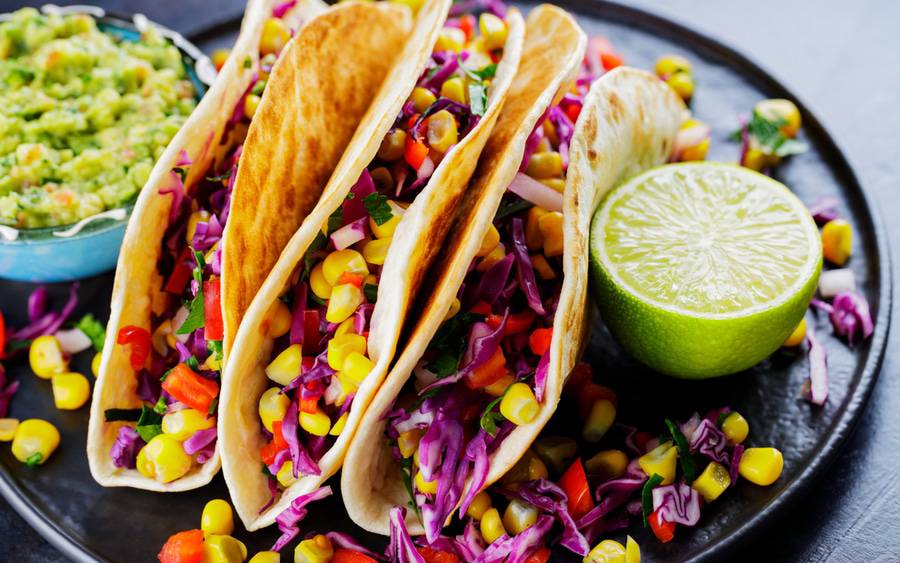The image features three golden-brown veggie tacos arranged on a black, cast iron plate. Each taco is made from crispy, fried corn tortillas and generously stuffed with vibrant ingredients. The fillings include yellow corn, diced red tomatoes, chopped purple cabbage, and finely diced green herbs likely to be cilantro. There is no visible meat in the tacos, suggesting they are vegetarian. Positioned on the right side of the plate is a half lime, cut and presented with the open face upward. To the left of the tacos and slightly above, sits a small blue bowl filled with guacamole, which is beautifully garnished with chunks of tomato. The ensemble creates a colorful and appetizing presentation.